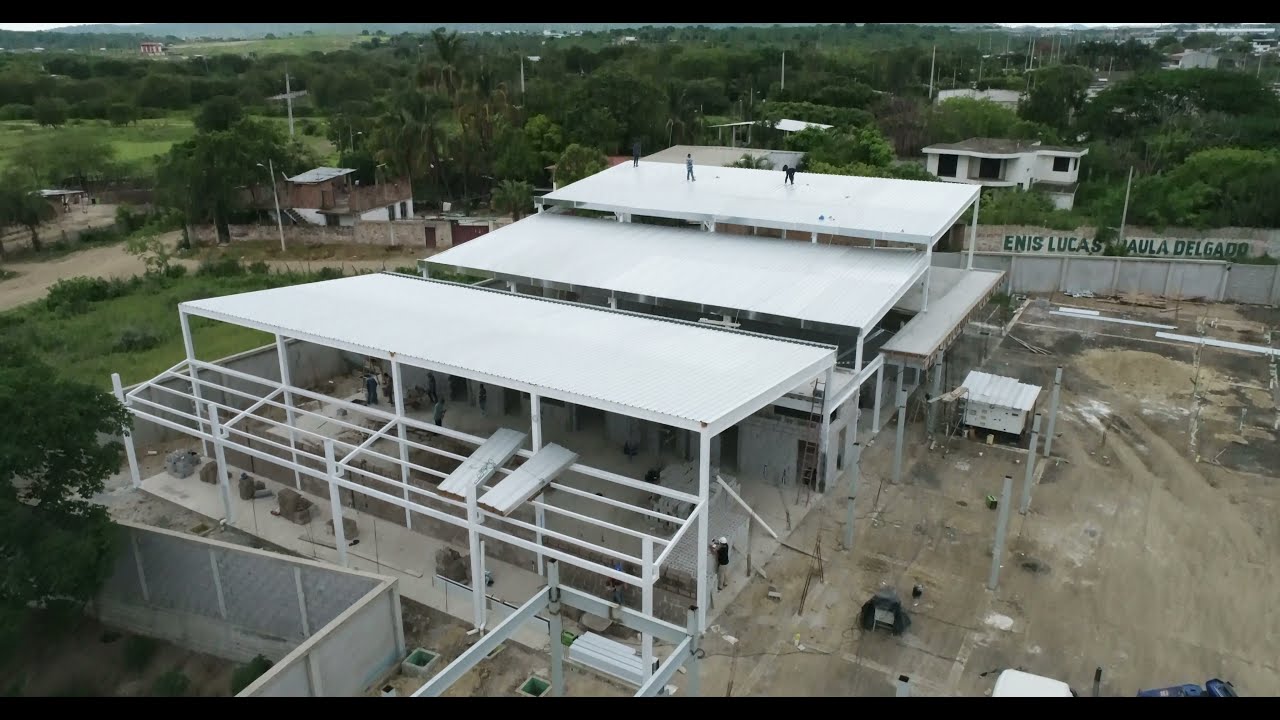The image depicts a sprawling, somewhat industrial or fairground-like area marked by a series of grayish-white, slightly sloping roofs supported by thin poles, reminiscent of structures common at a fair. The ground is covered in gray dirt and low grass, dotted with patches of grime. Prominently, in the center of the photo, there's a small, one-story building constructed from gray cement. This building connects to multiple white metal beams and tall awning-like roofs, creating mainly open but partially enclosed spaces beneath.

On the far right of the image, there's a visible sign reading "ENIS LUCAS AULA DELGADO," suggesting a Spanish context. People are seen both on the roof in the distance, likely engaged in some work, and on the ground beneath the first roof. The layout extends to reveal two additional awnings on the right side.

The top portion and left side of the image are framed by numerous trees, with a mix of natural elements such as grass and dirt roads peppered throughout. The far background features more trees and some houses, adding depth and context to the setting.